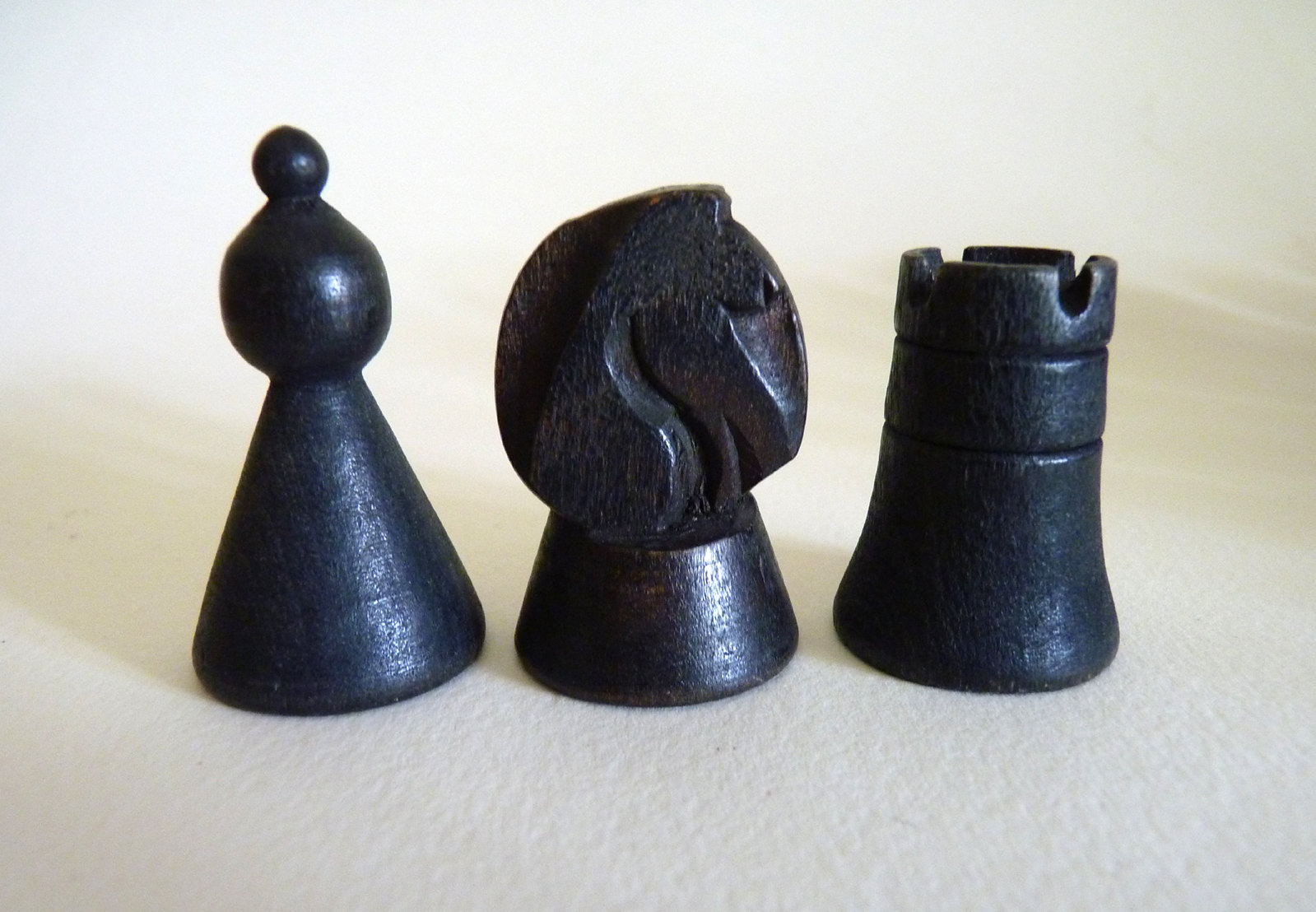This photograph showcases three intricately carved black chess pieces, likely made of stone such as granite or onyx. All the pieces rest on a white background, perhaps felt or cotton, casting subtle shadows around them. The piece on the left resembles a pawn, featuring a conical base with a bulbous top and a smaller ball perched above it. In the center, there is a stylized knight, or horse, with a distinct curved shape, although it's hard to identify definitively. The piece on the right is clearly a rook, structured like a castle turret. The white background and shadows add a dramatic effect, giving the impression that the pieces are part of an artistic display or museum exhibit, though their exact size remains uncertain as there is no scale reference in the image.